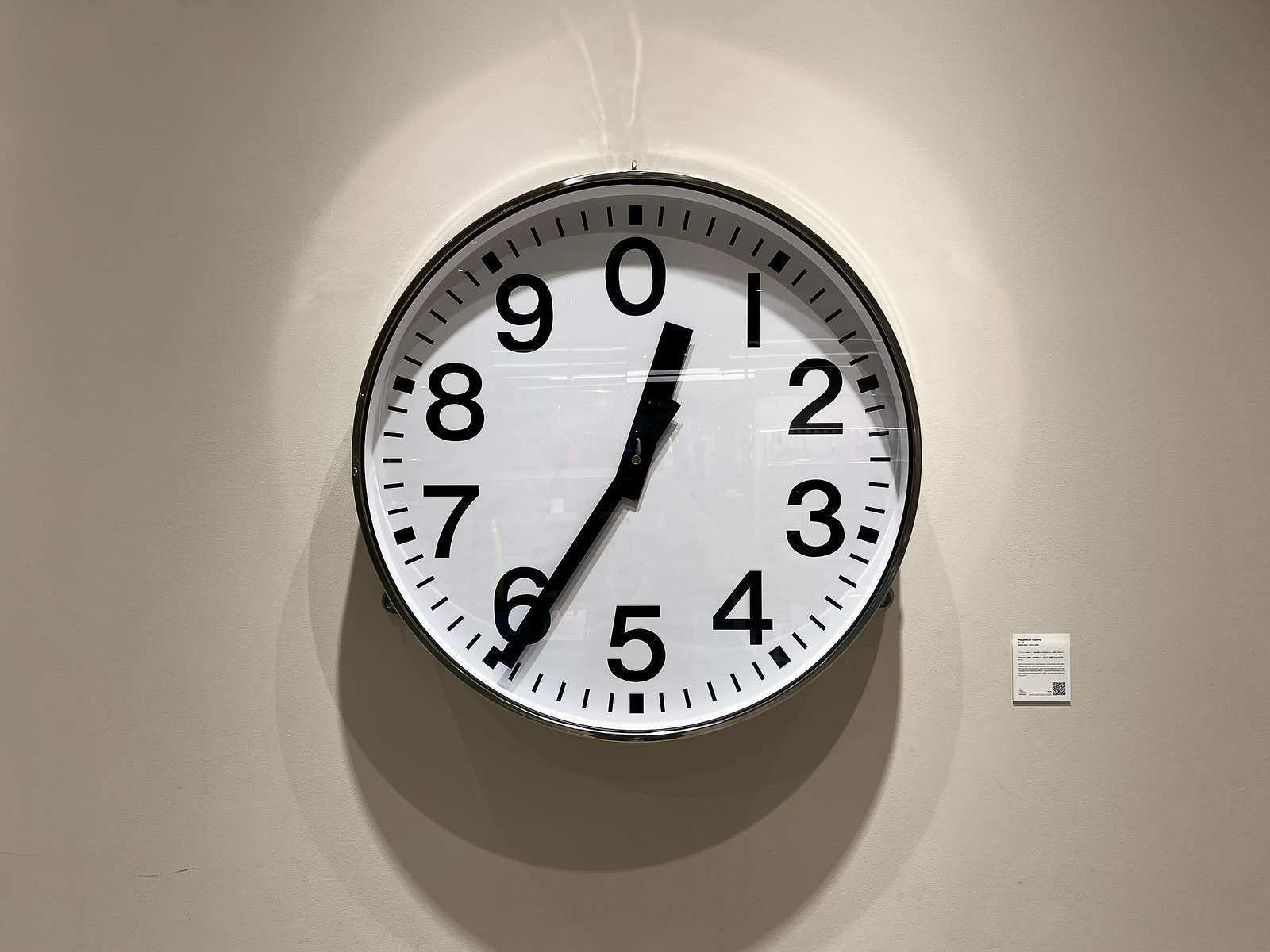The image features a photograph of a wall with a gray background, centered around a large, round clock with a black border. The clock has a white face with black numerals arranged in an unconventional sequence from 0 to 9. Nestled between these numerals are lines representing the minutes. Prominently displayed, the thick black hour hand is positioned between the 0 and 1, while the thick black minute hand is pointing at the 6. Below the clock, a shadow stretches downwards, mirroring its shape. In the lower right corner of the wall, there is a small, square-shaped item with illegible writing on it, potentially a label or sign. The clock’s unique numerical arrangement suggests it might be more of an art piece.